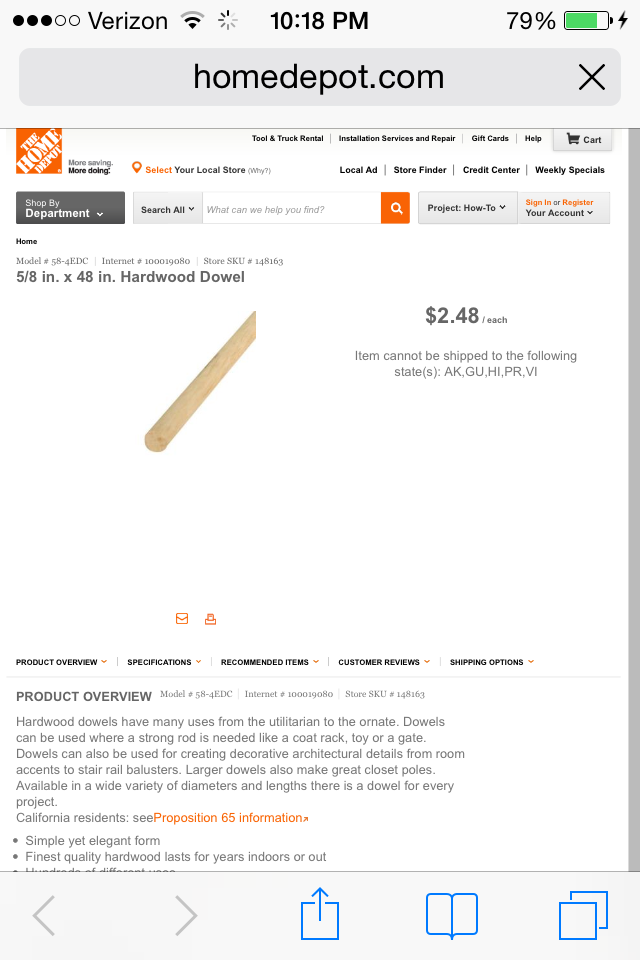The image is of a smartphone screen displaying a webpage from Home Depot on the Verizon network. At the top of the screen, there are three signal dots indicating the network strength, the time shown is 10:18 PM, and the battery life is at 79%. In the search bar, "homedepot.com" is entered. Below the search bar, the Home Depot logo is visible, followed by the words "Shop by Department" highlighted in gray.

Featured on the screen is a product listing for a "5/8 inch x 48 inch Hardwood Dowel," priced at $2.48 each. A notice informs that this item cannot be shipped to Arkansas, Guam (GU), Hawaii, Puerto Rico, and Virginia.

The product overview reads:
"Hardwood dowels have many uses from the utilitarian to the homemade. Dowels can be used when a strong rod is needed, like in a coat rack, toy, or gate. They can also be used for creating decorative architectural details, from room accents to stair rail banisters. Larger dowels also make great closet poles. Available in a wide variety of diameters and lengths, there is a dowel for every project. California residents see Proposition 65 information. Simple yet elegant form, first-quality hardwood ensures durability for years indoors and outdoors."

Navigation options at the bottom include a back arrow, forward arrow, share arrow, bookmark arrow, and a screen arrow.